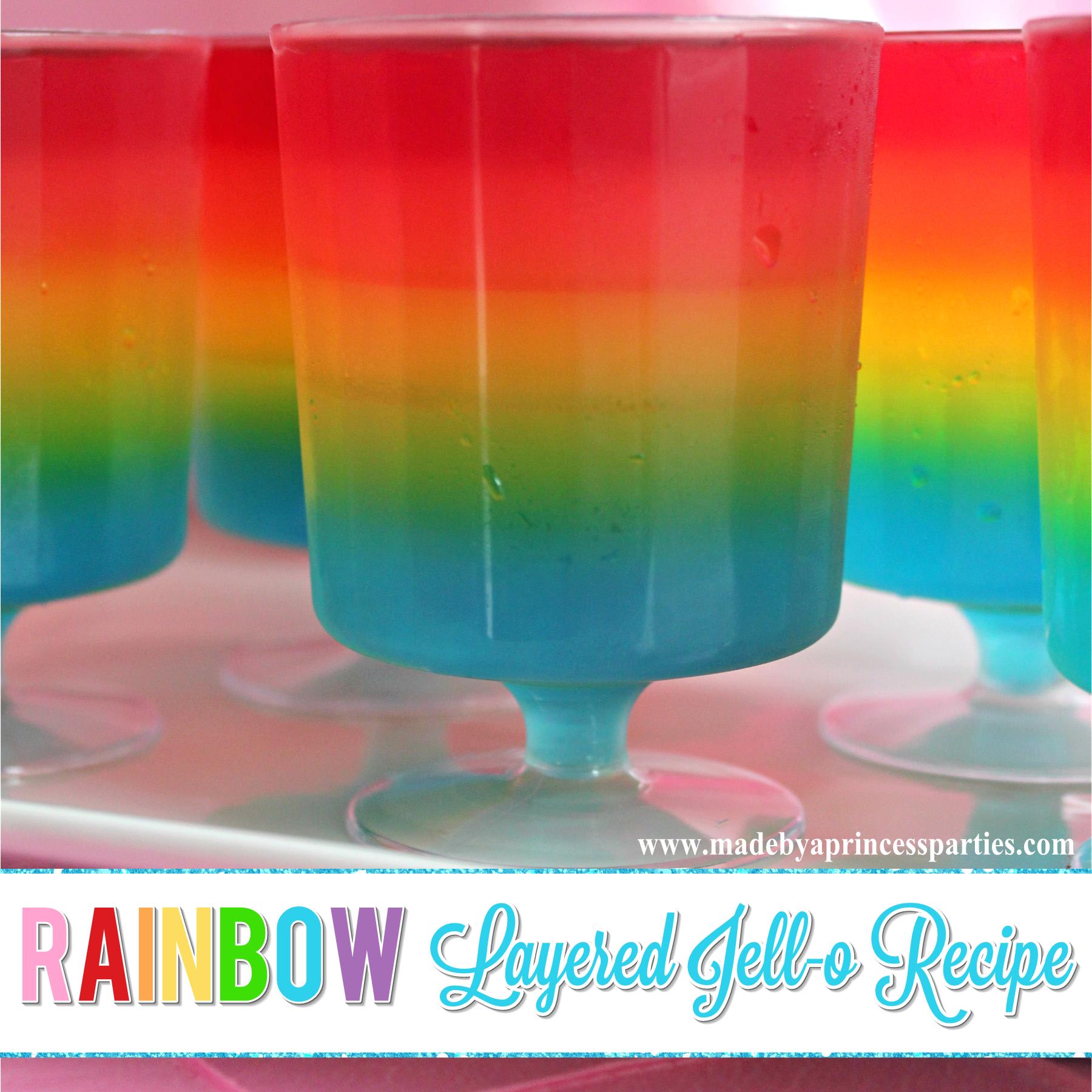This photograph showcases a visually striking setup of rainbow Jello parfaits, each meticulously layered in vibrant colors. At the bottom of the image, a pink line frames a prominent white rectangle, which is delicately outlined in light blue. Within this rectangle, the word "RAINBOW" is prominently displayed on the left side in bold, multicolored capital letters. To its right, the phrase "Layered Jello Recipe" is elegantly scripted in light blue cursive.

The center of the photograph features an array of glasses, each standing on a clear, circular base supported by a short stem, with the bowls flaring out gracefully. These parfait glasses are filled with precisely layered Jello, creating a captivating rainbow effect. Each glass is arranged with a dark red layer at the top, followed by a lighter red, then a vivid yellow, a bright green, and finally, a deep blue layer at the bottom. The central glass is surrounded by identical glasses, all showcasing the same rainbow-hued progression. This meticulous arrangement creates a visually delightful and colorful display that is both appetizing and aesthetically pleasing.